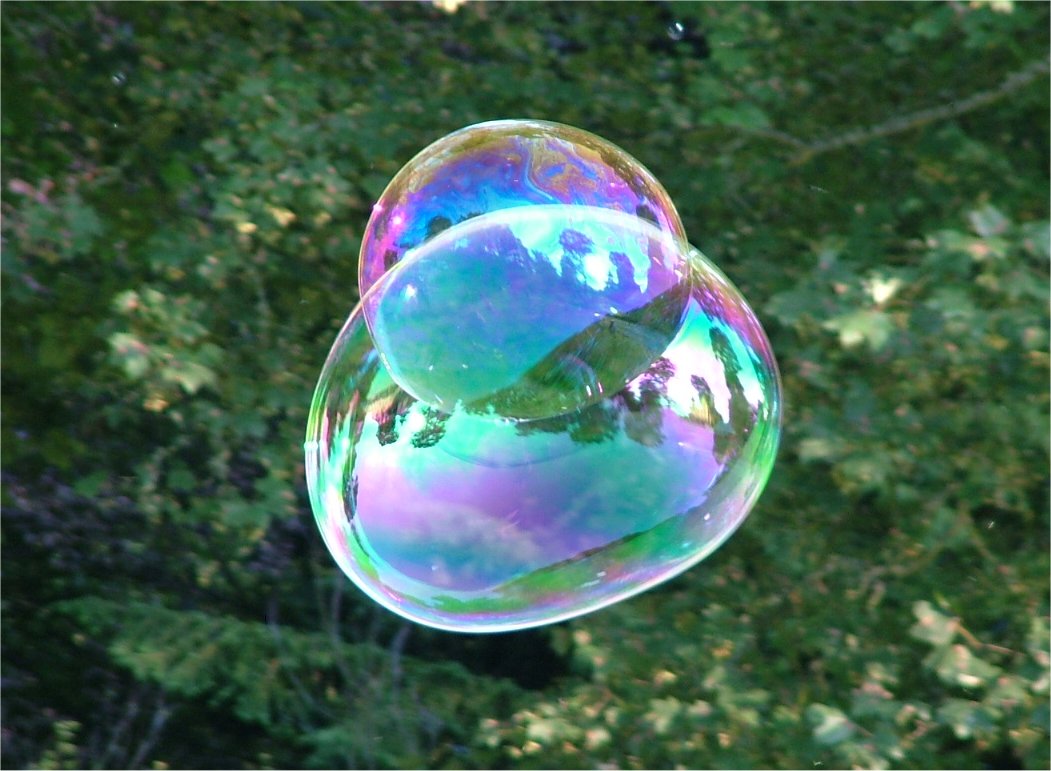A close-up photograph captures two large, shimmering soap bubbles floating amidst a lush, forested background. The dense foliage in the background features green leaves, with some tips shaded in brown, indicating they are slightly dried out. Thin, twig-like branches peek through the leaves, adding depth to the scenery. Amidst this greenery, a larger oblong bubble overlaps with a smaller, near-perfect spherical bubble, positioned towards the center of the larger one. 

Both bubbles exhibit a stunning translucent rainbow effect, reflecting a spectrum of colors including reds, blues, purples, oranges, and greens. The sunlight enhances their iridescence, making them appear very shiny. Notably, the bubbles mirror the surrounding landscape with the horizon line of trees and a cyan sky reflected within them, creating a captivating and surreal visual experience. The scene is serene and magical, with the bubbles floating gracefully above the tree line, suspended in a moment of natural beauty.